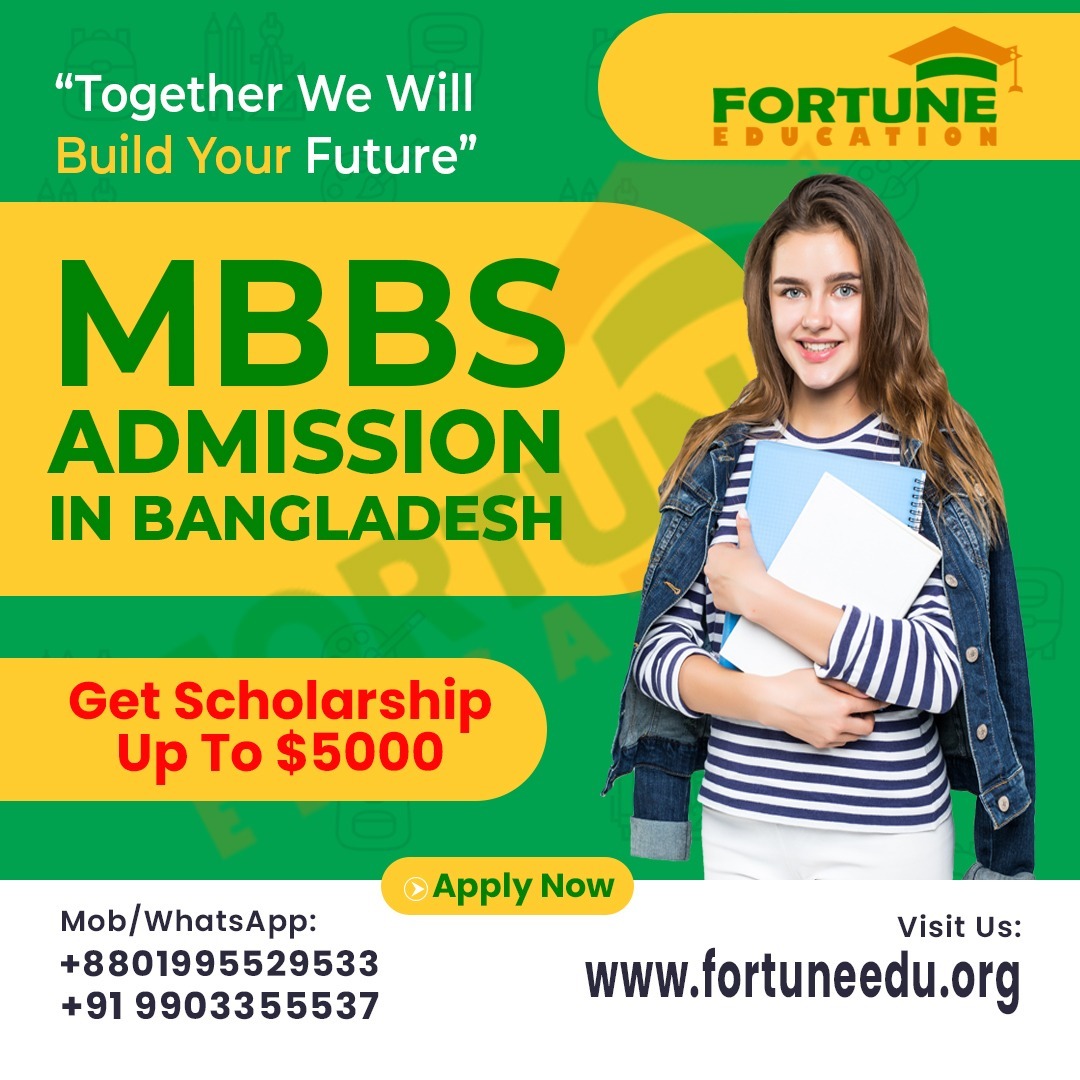The image is an advertisement promoting educational opportunities. At the top right corner, the ad displays the name "Fortune Education." Below it, the slogan "Together we will build your future" is featured prominently. The advertisement highlights an offer for "MBBS Admission in Bangladesh" with the potential to receive a scholarship of up to $5,000. For inquiries, the ad provides two contact options via mobile/WhatsApp at the numbers +8801995529533 and +919903355537. Centrally placed is a call to action, "Apply Now." On the lower right side, the ad directs viewers to visit the website at www.fortuneedu.org for more information.